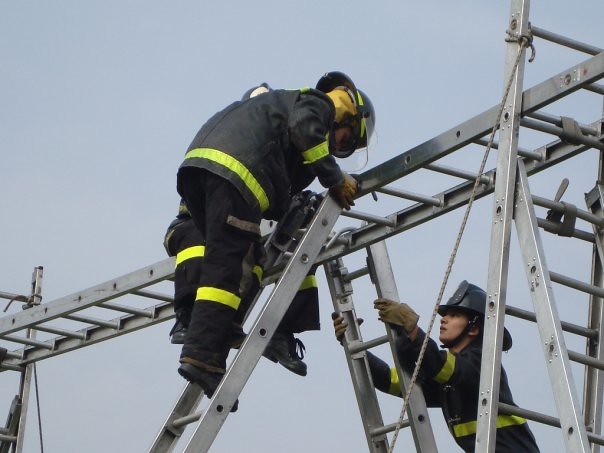This detailed photograph captures three firefighters engaged in what appears to be a training exercise involving chrome-colored ladders. The scene is slightly hazy, likely due to clouds or smog in the background. Two firefighters are actively climbing diagonal ladders, while a third firefighter can be partly seen, sitting astride a horizontal ladder, with only his legs visible. Each firefighter is clad in black and yellow gear, which includes black helmets, black jackets with yellow reflective stripes, black pants with matching yellow stripes, and black boots. Notably, one female firefighter at the bottom right corner wears brown gloves and holds the ladder for a middle firefighter. Both ladders are secured with ropes for stability, emphasizing the meticulous preparation and safety measures adopted during the exercise. The ladders are the sturdy, stainless steel type commonly used by firefighting professionals.